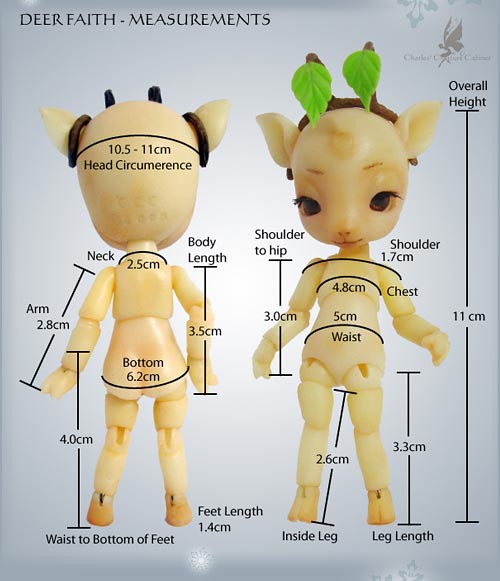The image depicts a detailed diagram of a doll named "Dear Faith Measurements" against a light blue background. The doll, which is a blend of a humanoid and a deer, is shown from both the front and back perspectives. The cream-colored doll has a face resembling a baby deer, complete with pointed ears and a headband featuring two green leaves. The measurements of various parts of the doll's body are meticulously labeled in black text, with indications for overall height (11 cm), shoulder to hip (3 cm), waist (5 cm), chest (4.8 cm), shoulder (1.7 cm), inside leg (2.6 cm), leg length (3.3 cm), feet length (1.4 cm), waist to bottom of feet (4.0 cm), neck (2.5 cm), body length (3.5 cm), bottom (6.2 cm), and arm (2.8 cm). The background includes subtle white and light gray snowflakes at the top right and bottom corners. This thorough depiction helps provide a comprehensive understanding of the doll's proportions.